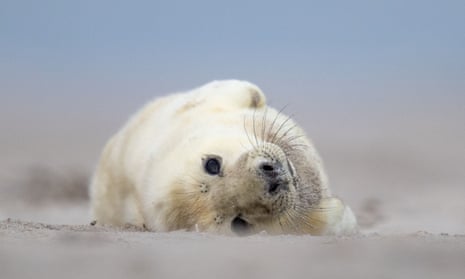This photograph captures a close-up view of a baby seal pup lying on its side, seemingly in a snowy or icy environment. The seal, likely a gray seal, has an endearing presence with its fluffy white fur, accented by beige patches around its snout and head. Its dark, expressive eyes and pitch-black nose stand out vividly, complemented by black whiskers around its mouth. The seal's flippers are tucked close to its body, one visible on top and the other beneath it. It is positioned at the center of the image, with its body slightly rolled showing its belly on the right and back on the left. The background is a blur of gray, white, and blue hues, creating a soft-focus effect that makes it hard to distinguish the sky from the ground, yet contributing to the serene and tranquil feel of the setting. The seal appears relaxed, gazing directly at the camera, making it the focal point of this charming and peaceful scene.